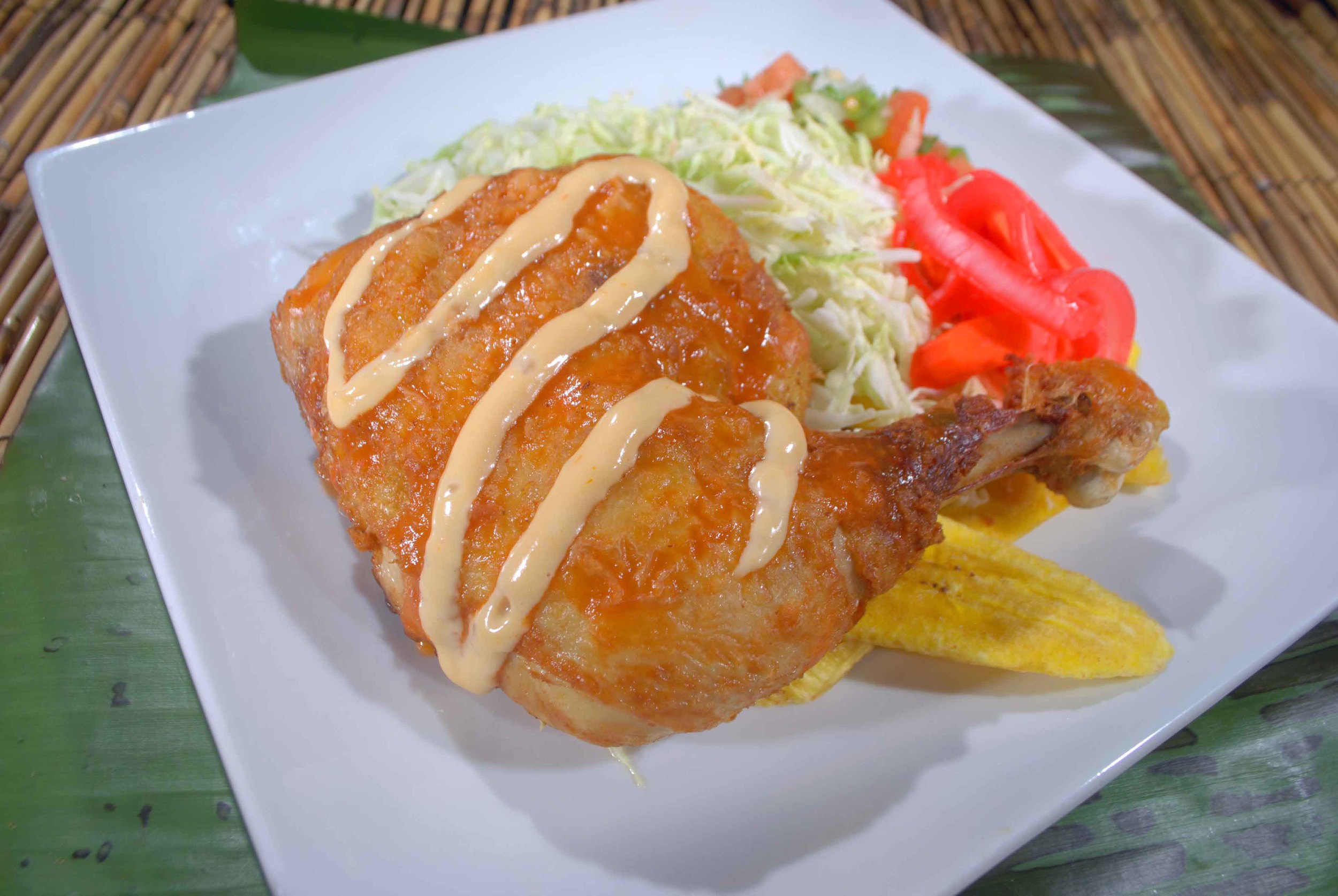The image captures a plated meal set in a likely restaurant setting. The focal point is a white square plate, slightly tilted, placed on a green banana leaf serving as a placemat, atop a rustic wooden or bamboo table. The center of the plate showcases a golden-brown chicken wing or leg piece, drizzled with a zigzagging pinkish sauce, which might be a variant of mayo or a light cream sauce. Surrounding the chicken, there is a vibrant mix of shredded green lettuce or cabbage, red tomato pieces or red onion slices, and yellow plantain or papaya slices. The arrangement is visually appealing and hints at a delicious and well-rounded meal.